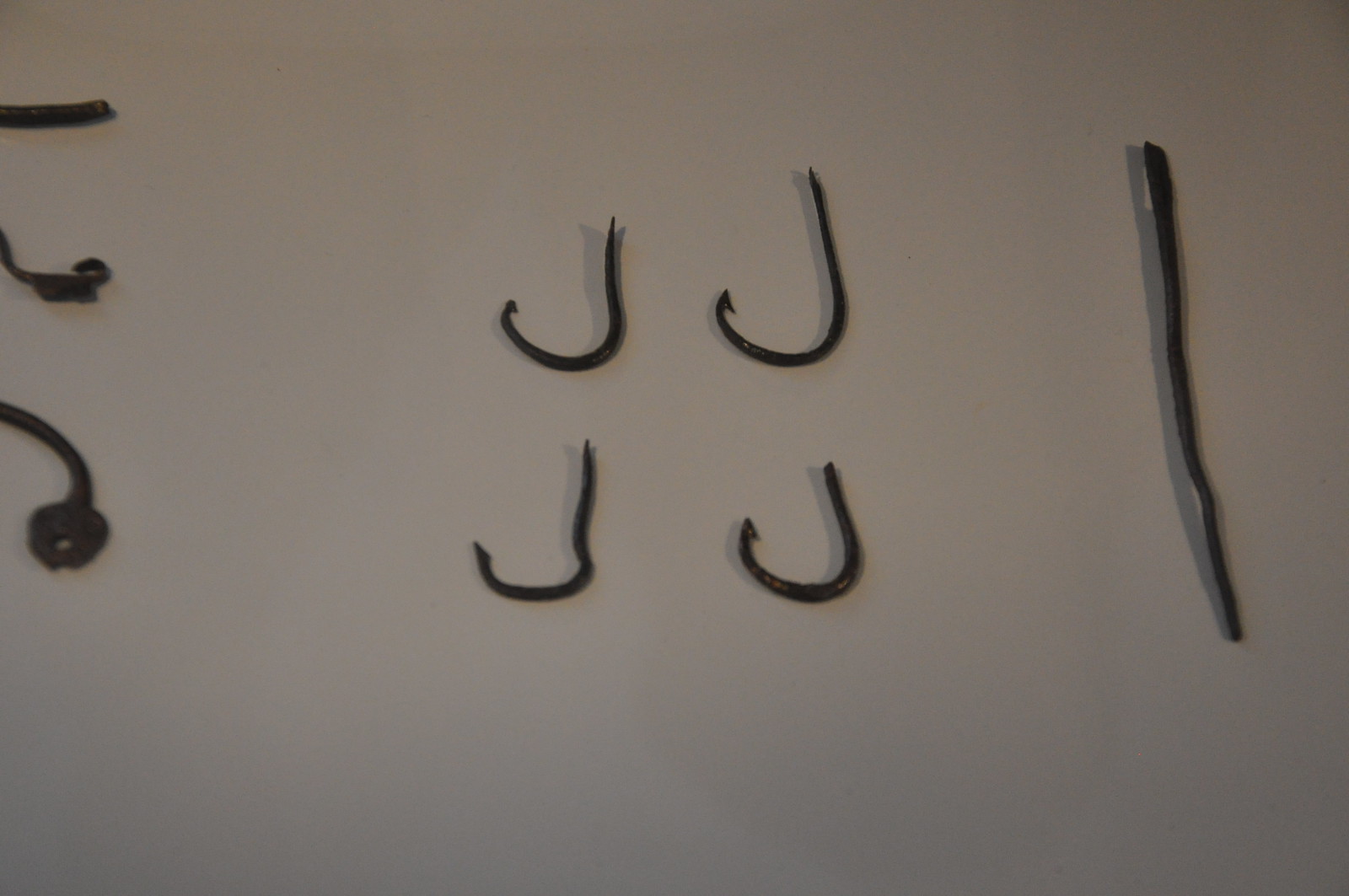The image depicts a top-down, darkly-lit scene with a gradiated brown to grayish-brown background. In the center lie four antiquated, black metal fish hooks, some larger and some smaller. The bottom left hook is notably almost square-shaped at its base, deviating from the typical rounded form. All four hooks cast gray shadows to their left. Surrounding the hooks are other indistinct black metal pieces; to the left, the irregular fixtures are partially obscured, and to the right, there is a slightly bent black metallic shaft or spike. The details suggest the hooks and metal items are aged, possibly museum artifacts, set against an indoor, softly illuminated background.